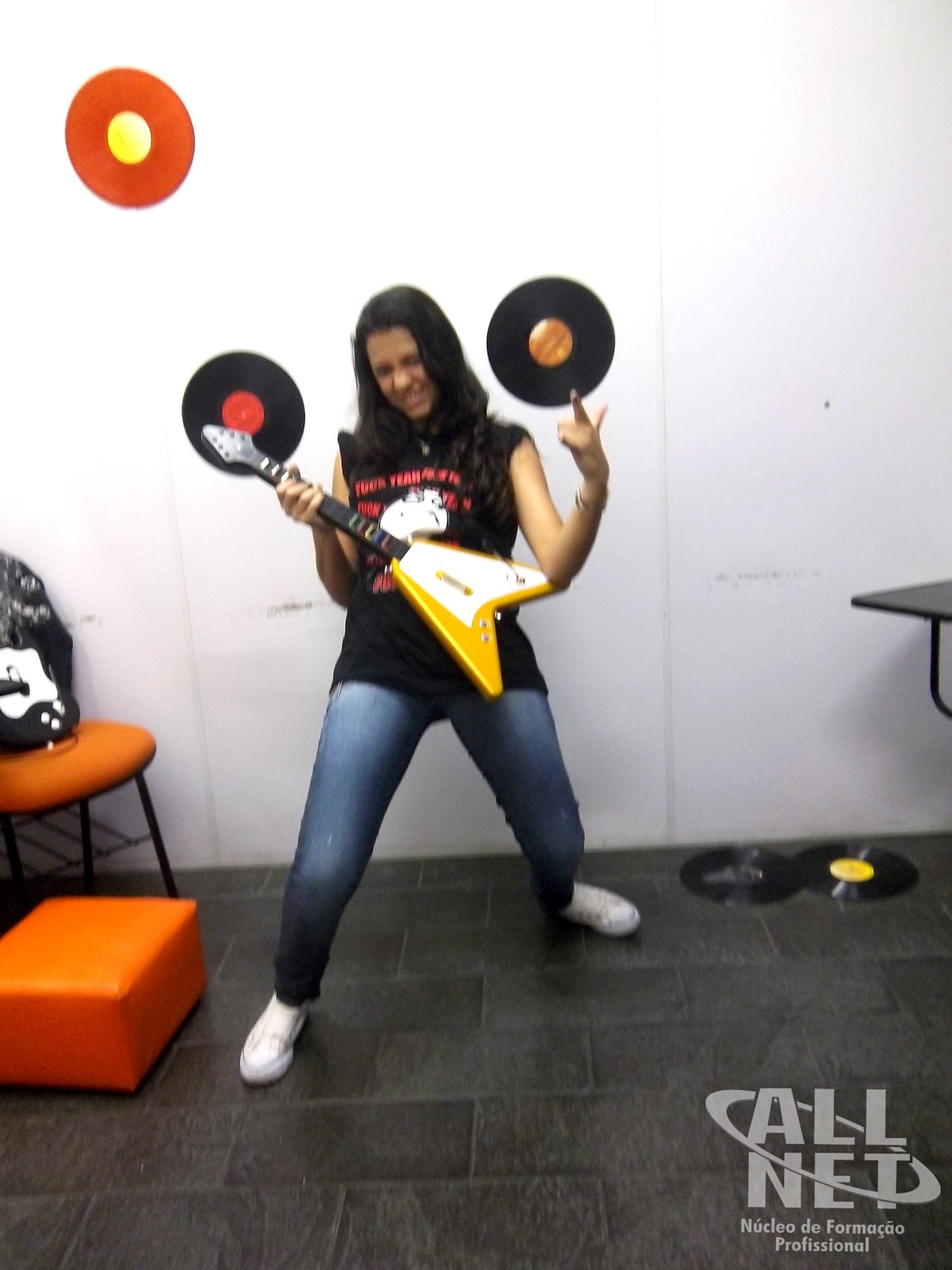In this image, a woman is posed as a rock star, enthusiastically holding a toy guitar similar to those used in video games like Guitar Hero. She's wearing a black t-shirt with white and red accents, light blue jeans, and white sneakers. The guitar features a striking gold, white, and black color scheme, with a distinctive triangular body marked by a white pickguard area and yellow wood detailing. She stands in a dynamic power stance, her right foot forward, while her left hand points skyward, and her right hand grips the guitar neck.

Her eyes are closed, and she wears a joyful smile, embodying the spirit of rock 'n' roll. The background of the image includes a white wall adorned with several records: two black records positioned near her head and a red record in the top left. The floor is dark gray, and the foreground includes an orange chair and matching footrest with black legs on the left side, along with more records scattered on the floor to her right.

At the bottom right corner, text reads, "All Net Nucleo de Formacio Proficional," indicating a possible Spanish or Portuguese professional training center. The overall scene captures the playful energy and fun of the moment.